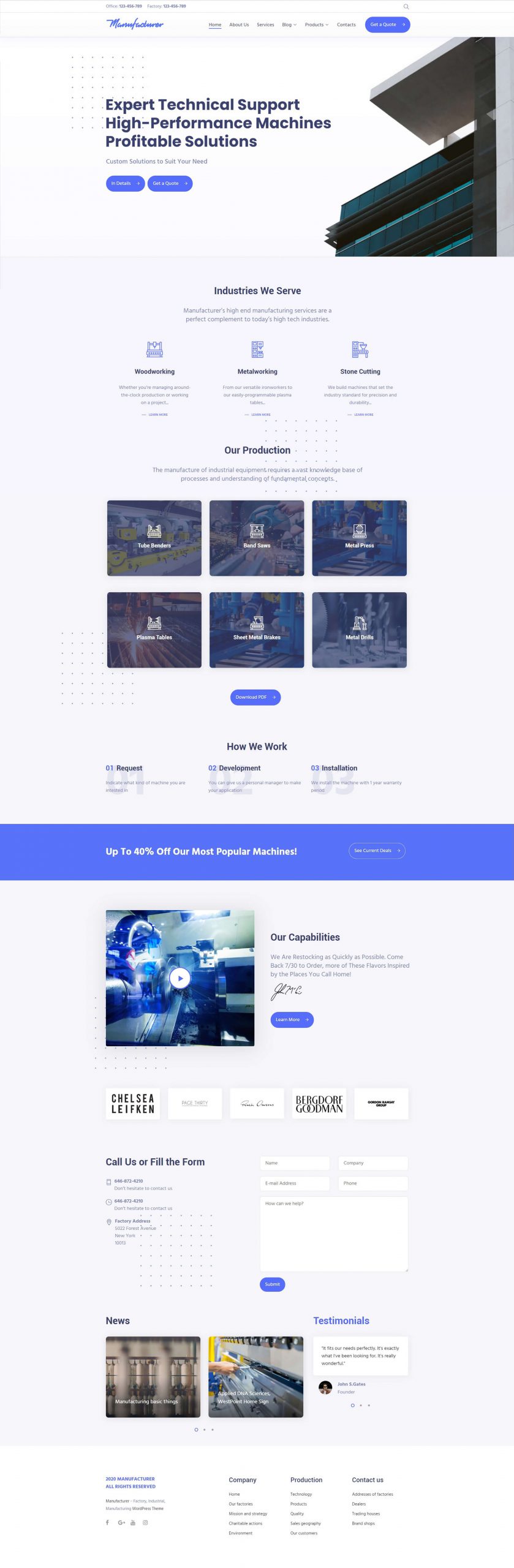The image is blurry, but some details are discernible. At the top of the image, there is a heading written in dark blue text that reads "Expert Technical Support, High-Performance Machine, Profitable Solution." Below this heading, there are two blue buttons that are not clearly visible. Further down, the text "Industries We Serve" appears, followed by the names of various industries which are not readable. 

Another section titled "Our Production" is visible, detailing features across six different parts, though the text is illegible. Following this is a segment titled "How We Work," featuring an explanation that is also unreadable. Near the bottom, there is an offer stating "Up to 40% off our most popular machines." The background for this text is blue, while the rest of the image background remains white. 

Towards the bottom, the name "Chelsea Leifkea" is displayed. Below this, there is a section called "Our Capabilities," though the text here is also not legible. The image also includes forms or links with instructions to "Fill the Form" on the left side, a "News" section, and "Testimonials" written in blue text positioned in the bottom right corner.